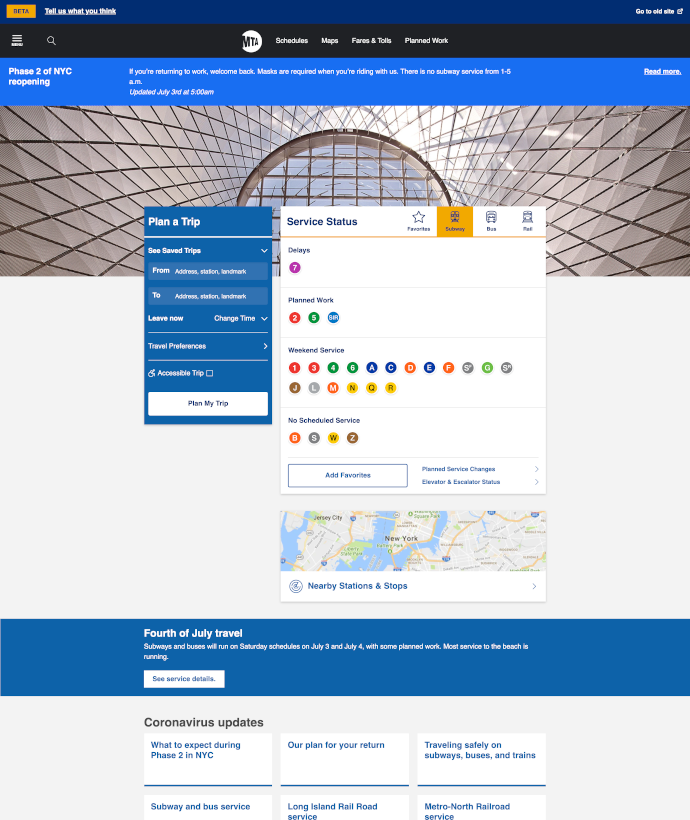This image showcases the beta version of the New York Metro Transit Authority's website. The interface features a dark blue horizontal banner at the top, with a yellow 'Beta' label situated in the upper left corner. Adjacent to it is a prompt encouraging visitors to "Tell us what you think." On the upper right corner, there’s an option to "Go to old site" accompanied by a clickable button for redirection.

Beneath the top banner, a black horizontal navigation bar spans the page. It includes a menu option on the far left, a search bar next to it, and at the center, the MTA logo. To the right of the logo are navigational links labeled "Schedules," "Maps," "Fares and Tolls," and "Planned Work."

A blue horizontal banner located below the navigation bar announces "Phase 2 of NYC Reopening" with a welcoming message for those resuming work, reminding them that masks are mandatory when using the transit system. The banner also notifies users of the subway service suspension from 1 to 5 a.m., with an update timestamped July 3rd at 5 a.m. It concludes with a "Read More" link on the far right for additional information.

Further down the page, the background features an impressive photograph looking up at a domed glass ceiling. Centered on the page is a "Service Status" box, and beside it, to the left, is another box designated for "Planning a Trip." At the bottom of the page, there are updates about 4th of July travel and the latest information on coronavirus measures.